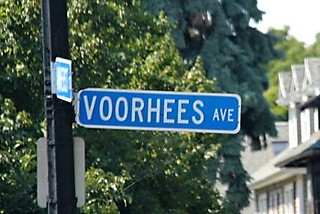This photograph, taken on a clear day, prominently features a street sign on a black metal pole. The blue rectangular street sign reads "Voorhees Avenue" in all-capital white letters, bordered in white. Above the street sign, there is a blue sticker with the letter "E." Behind the pole, a variety of green trees provide a lush background, showcasing different shades and leaf types. To the left and right of the pole, the tops of white and brown houses are partially visible, with distinct peaked and porch roofs. In the right section of the image, a white house with posts, windows, and dormers can be seen. A bit of white sky is visible in the upper left corner, completing the outdoor scene.